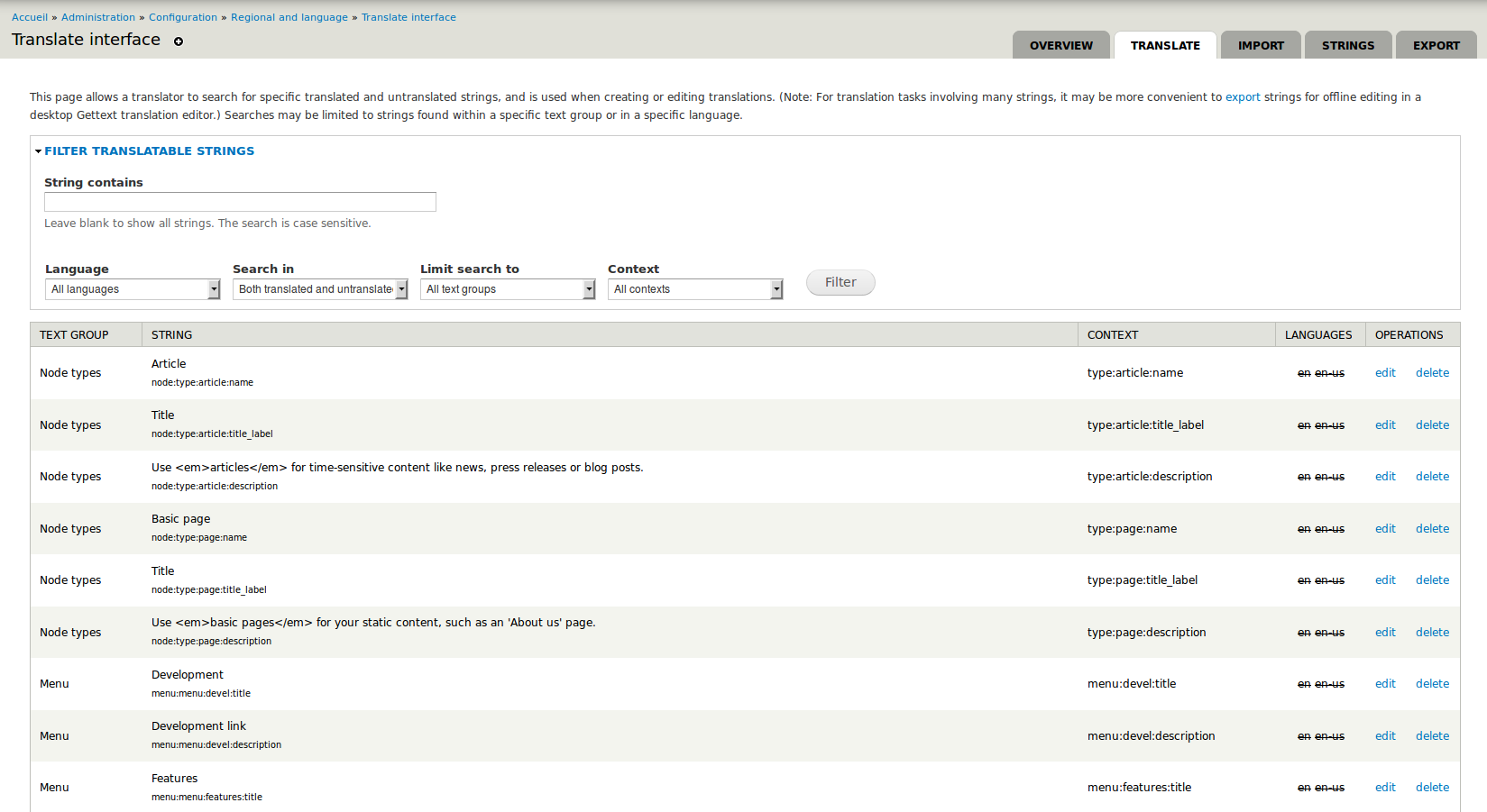An image taken from a digital screen displays an interface labeled "Translate Interface" at the top. Just above this, in blue text, is "ACCUEIL." Below it, tabs read "Administration," "Configuration," "Regional and Language," and "Translate Interface." 

The main section features a detailed instructional note: "This page allows a translator to search for specific translated and untranslated strings, and is used when creating or editing translations." A parenthetical note adds: "Note: For translation tasks involving many strings, it may be more convenient to export strings for offline editing in a desktop Gettext translation editor. Searches may be limited to strings found within a specific text group or in a specific language."

The interface includes a search option labeled "Filter Translatable Strings." Below this, a list itemizes various node types and their properties, including "Article," "Node Type" (with multiple entries like "Title" and "Use"), "Basic Page," and "Development Link." Additional listed features progress further down the screen.